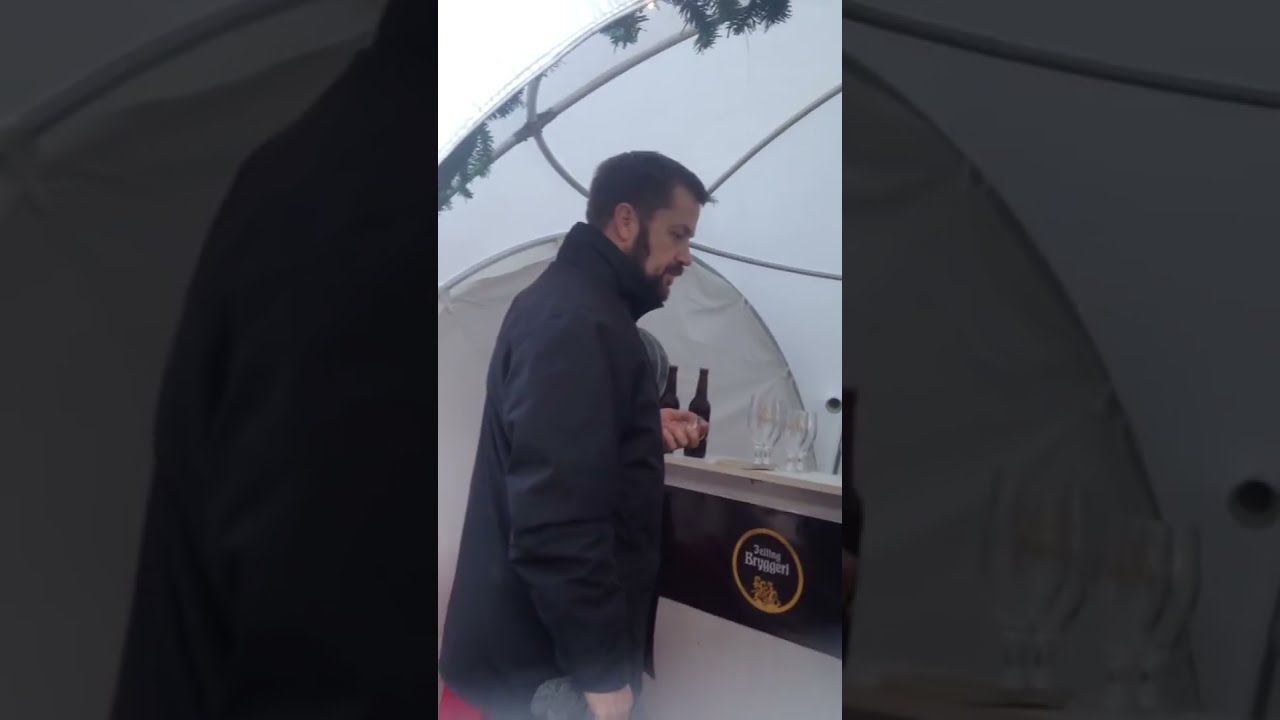In the image, there is a man and a woman inside a dome-shaped white tent, which resembles a festival pavilion. The man, seen from the side profile, has short light brown hair and is wearing a vibrant plaid shirt with shades of blue, yellow, and red, along with a dark woolen scarf and gray gloves. He is holding a large, shiny black bottle with a brightly colored label adorned with yellow, red, and white text, turned away from the camera, making the details of the label hard to decipher. The man appears to be presenting this bottle, perhaps indicating a demonstration or promotional display. Beside him, the woman with a ponytail and substantial makeup is looking at him with a blank expression. She is visible from the shoulders up, presumably wearing a coat given the cold setting suggested by their attire. In front of them, there is a desk with a plain white surface, a few glasses, and what appears to be a dark logo. The interior of the tent shows the wire framework supporting the structure overhead.